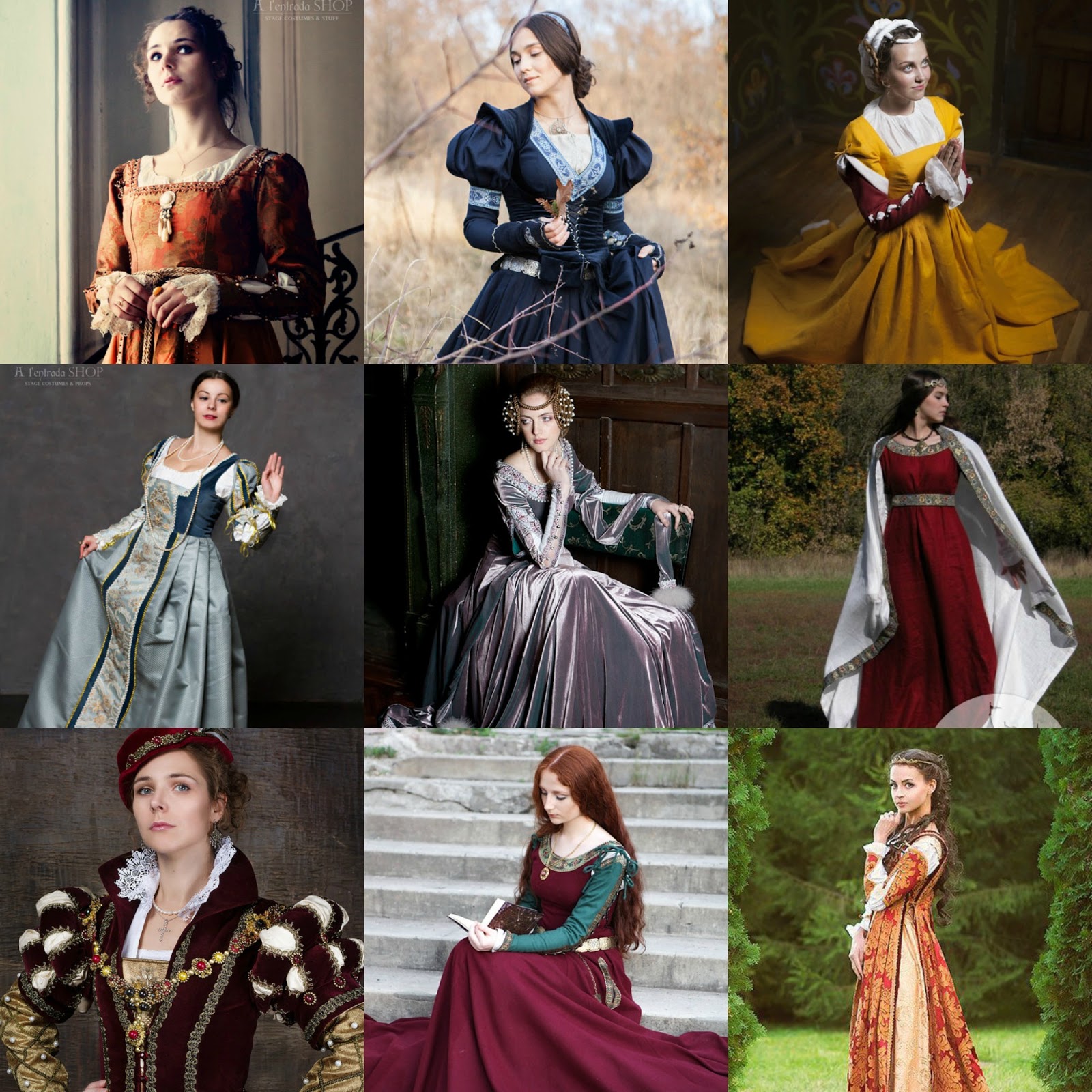The image is a detailed photo collage consisting of nine individual photographs arranged in three rows of three, each featuring a young woman dressed in elaborate, historical-style gowns suggestive of medieval or olden times attire. The women are predominantly Caucasian with dark hair, except for one redhead. The dresses displayed are characterized by voluminous skirts and fitted bodices typical of their era.

In the upper left, a woman with brown hair and a flowing red dress appears, while next to her, another brown-haired woman in a dark blue dress stands amidst a wooded area. At the top right, a woman in a white and yellow dress is kneeling as if in prayer, adorned with a white headdress. 

The middle row begins with a woman dressed in a blue and yellow gown against a gray background. At the center of this row, a woman in a silvery gown with a brown headdress is seated, and to her right, another woman in a white robe or cape stands out.

The bottom row starts with a woman in a red, fluffy gown reminiscent of a 17th-century royal uniform. In the middle, a red-haired woman in a magenta dress sits on steps, engrossed in a book. The final image on the bottom right features a brown-haired woman in a floral yellow and red dress, posed amidst green trees.

The settings of the photographs vary, with some women indoors while others are pictured outside in fields, gardens, or wooded areas.